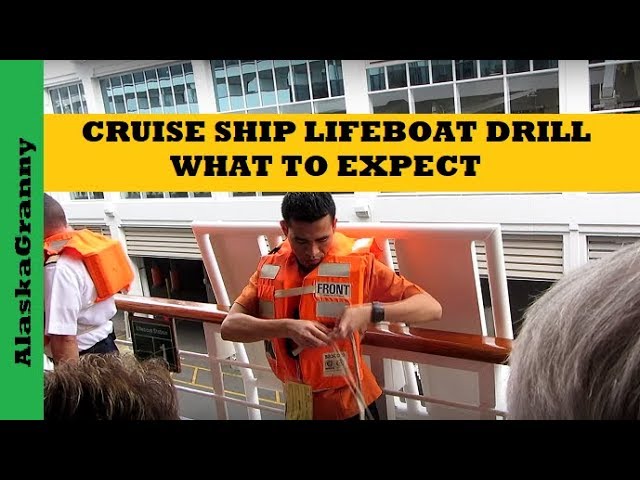The photograph captures a detailed scene of a man, likely a crew member, standing on the deck of a cruise ship conducting a lifeboat drill. The man is positioned centrally in the image and is wearing an orange life vest while demonstrating how to secure it. Behind him, the side of the cruise ship is visible, complete with windows. The audience, consisting of the partially visible heads of two individuals—one with white hair and the other with brown hair—observes the demonstration from the lower corners of the photo. Additionally, the back of another crew member, also dressed in an orange life vest, is visible in the center-left portion of the image. Above the scene, a yellow horizontal banner stretches across the top of the photograph, bearing the text "CRUISE SHIP LIFEBOAT DRILL: WHAT TO EXPECT" in bold black letters. Along the left border, a green vertical strip reads "ALASKA GRANNY" in black letters, oriented from bottom to top. The photo is framed with black borders at the top and bottom, emphasizing the importance of the drill being conducted.